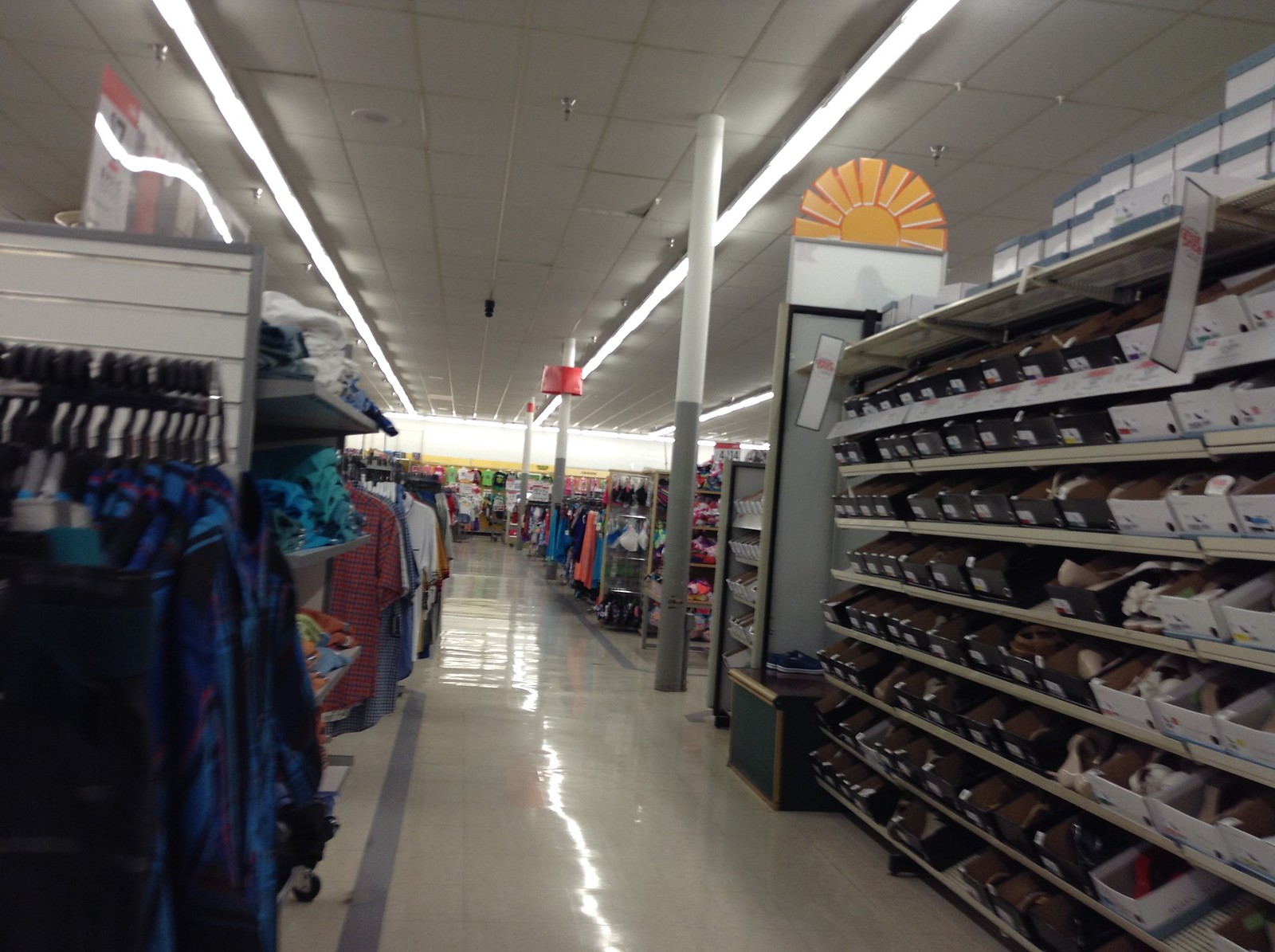The image captures the interior of an old and somewhat outdated department store, possibly a retail store like Kmart. The scene is set in a main aisle with glossy linoleum flooring featuring white tiles accented by gray edges and blue strips. Flanking the aisle on the right are numerous racks filled with shoe boxes, predominantly in black, white, and gray. Notably, the lids of many boxes are open, inviting customers to inspect the shoes inside. On the left side, a variety of clothing is displayed on hangers, including blue, red, and white shirts, as well as blue and black flannel plaid shirts. Toward the top of the aisle, conspicuously stands a square sign adorned with a sun-like symbol. Further back, structural gray and white poles support the ceiling, which is outfitted with long, white fluorescent lighting strips.